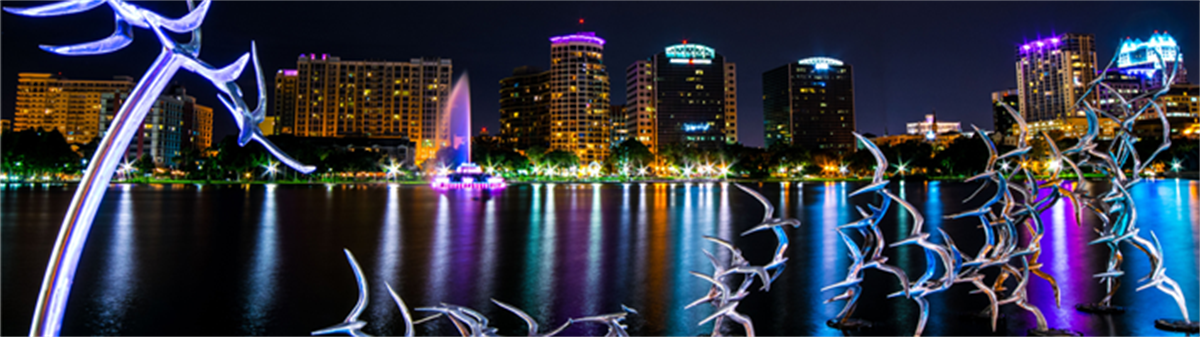The image captures a vibrant cityscape at night, resembling downtown Miami with its rich array of neon colors. The scene features six or seven prominent high-rise buildings illuminated in shades of purple, blue, orange, and green. These vibrant hues reflect off a body of water in the foreground, creating a mesmerizing mirror effect. The shoreline is also lined with bright lights, possibly from passing traffic, which add to the lively atmosphere. The night sky is dark, accentuating the luminous city. In the foreground, there appears to be a structure depicting birds—possibly seagulls or doves—flying in a flock. These birds, which may be superimposed and have a crystalline or metallic appearance, add an intriguing artistic element to the image. One building stands out on the right side, crowned with a striking neon blue light, further enriching the scene's colorful palette.